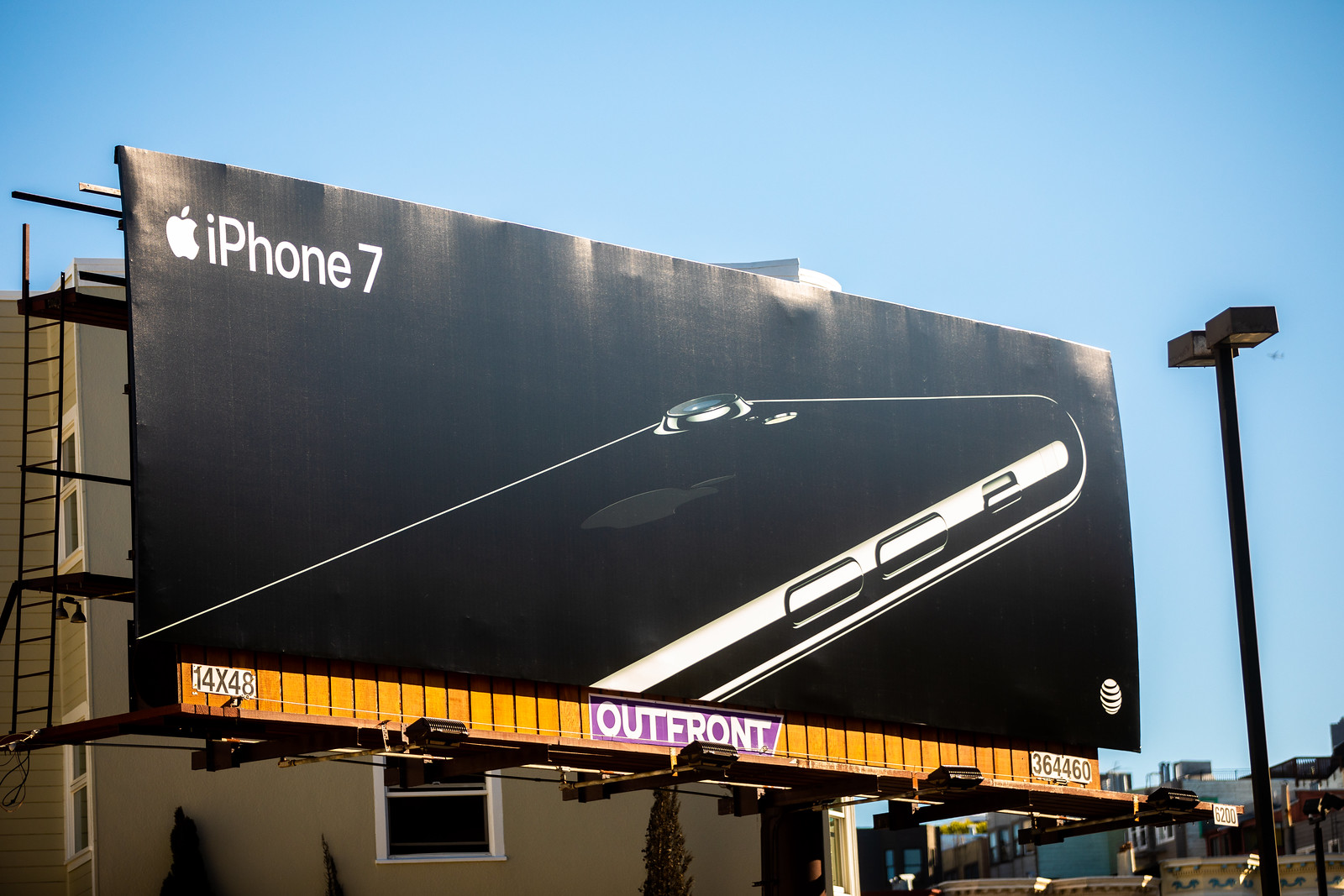This outdoor photograph focuses on a large, predominantly black billboard set against a bright blue sky. Dominating the upper left corner of the billboard is the Apple logo alongside the text "iPhone 7" in white. The central portion of the billboard features a close-up image of the iPhone 7, emphasizing its sleek, black, and reflective design. In the lower right corner of the billboard, the AT&T logo is displayed in black and white. Below the main advertisement, an orange strip stretches across the bottom with the dimensions "14 by 48" on the left, a purple section in the center reading "Out Front," and the numbers "364460" on the right. Behind the billboard stands a grayish building with a single window, flanked by green, pointy shrubs. To the right side of the billboard, a black streetlight with two square lights at the top is visible. The scene is framed by a cityscape of low buildings, enhancing the urban outdoor setting.